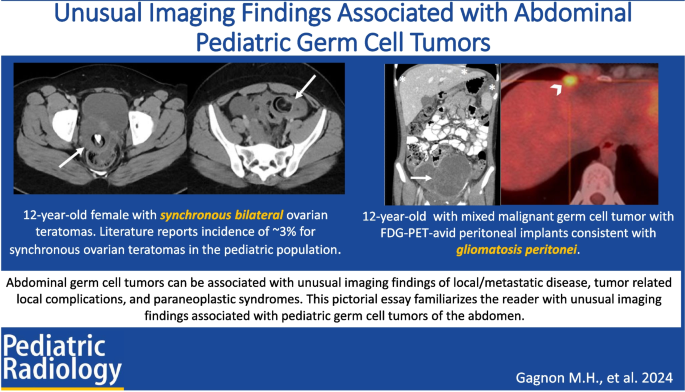The image appears to be sourced from an academic journal, specifically the Pediatric Radiology journal, as indicated by the label in the bottom left corner. The heading at the top reads, "Unusual imaging findings associated with abdominal pediatric germ cell tumors" on a white background in black text.

Below the heading, the presentation features a blue background with two distinct imaging slides positioned side by side. On the left, there's an image of a 12-year-old female diagnosed with synchronous bilateral ovarian teratomas, highlighted with white, grey, and black hues along with arrow markings pointing to specific areas. The accompanying text notes that the incidence of synchronous ovarian teratomas in the pediatric population is less than 3%.

On the right side, the slide includes a mixed image showing both grayscale and color. The grayscale portion depicts the liver and other organs, while the color portion highlights the liver in red with yellow dots. This image corresponds to a 12-year-old with a mixed malignant germ cell tumor and FDG-PET avid peritoneal implants, consistent with gliomatosis peritonei.

Below these images, text on a white background further elaborates that abdominal germ cell tumors can exhibit unusual imaging findings, including local metastatic disease, tumor-related local complications, and paraneoplastic syndromes. The pictorial essay aims to familiarize readers with these initial imaging findings associated with pediatric abdominal germ cell tumors. The authors of the study are listed in the bottom right corner as Gagnon M.H. et al. 2024.